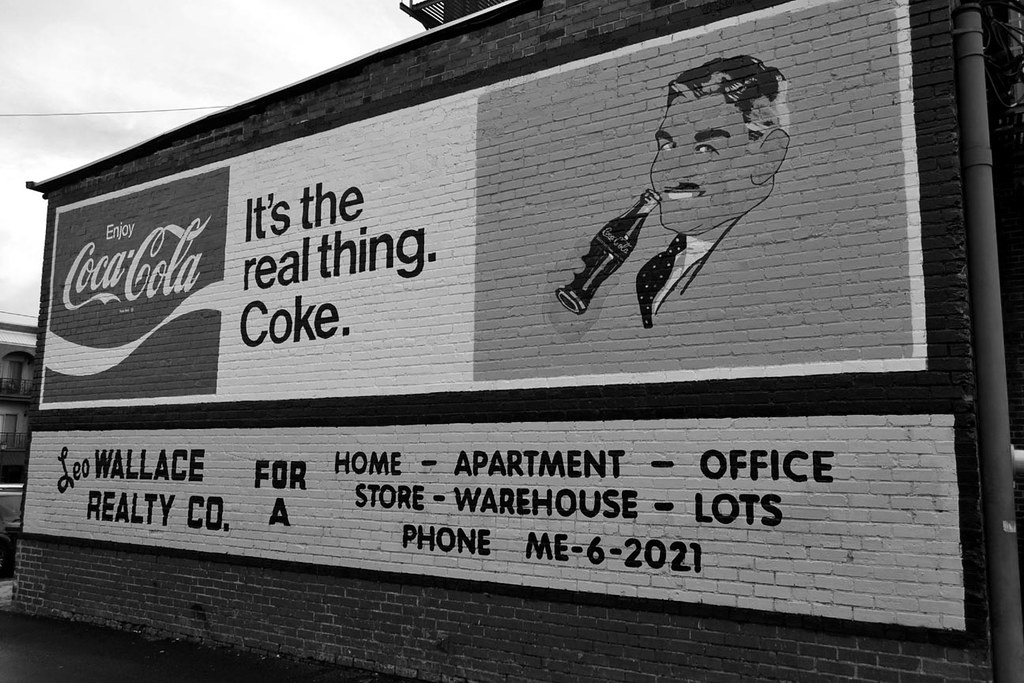The black-and-white photograph captures the side of an old building with a weathered brick wall adorned with a vintage Coca-Cola advertisement and a realty sign. The upper portion of the wall prominently features the distinctive, cursive Coca-Cola logo with a white ribbon beneath it. Adjacent to the logo, a white panel displays the phrase "It's the real thing, Coke" in black letters. To the right, a grayscale illustration depicts a mustached, middle-aged man enjoying a bottle of Coca-Cola. Below this advertisement, painted directly on the bricks, is a white rectangular panel with black text: "Leo Wallace Realty Co. for home, apartment, office, store, warehouse, lot, phone me 6-2021." The backdrop captures a light sky, adding to the nostalgic ambiance of the scene.